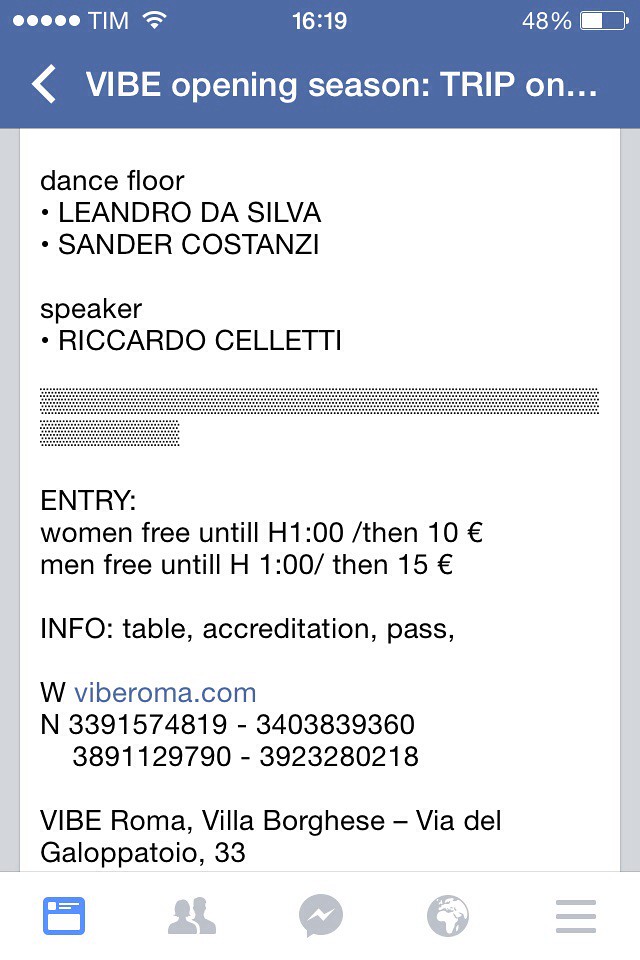The image depicts a rectangular screenshot from a cellphone screen, identifiable by the blue status bar at the top displaying the time, battery level, and signal strength. The focal content is an email, announced with the bold heading "VIBE OPENING SEASON TRIP," which is partly truncated. Below this are the details of the event against a white background in black text.

The event details are structured as follows:
- "Dance Floor" followed by the names Leandro Da Silva and Sander Costanzi.
- "Speaker" listed as Ricardo Soletti.
- A dividing bar that states the entry fees: "Women free until 1:00, then €10" and "Men free until 1:00, then €15."
- Further information including "Info, table, accreditation, pass."

Additional contact details provided include a website URL, Viberoma.com, and phone numbers, along with an address at the bottom: "Viberoma, Villa Borghese, Villa del Galapetillo 33."

The screen also displays common mobile interface icons at the bottom, including options to save, access contacts, and messaging functions.